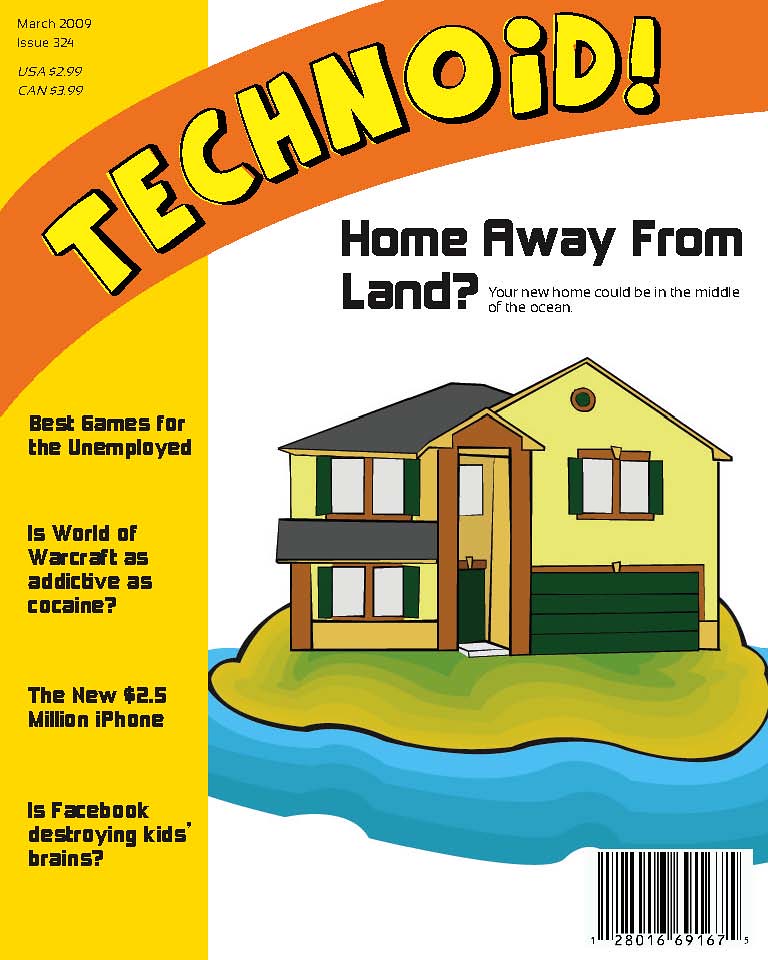The cover scan of the magazine "Technoid!" dated March 2009, Issue 324, priced at $2.99 in the USA and $3.99 in Canada. The magazine title "Technoid!" is prominently displayed in large, yellow, cartoonish letters against an orange background. A yellow band on the upper left contains black text listing various feature stories: "Best Games for the Unemployed," "Is World of Warcraft as Addictive as Cocaine?" "The New 2.5 Million Dollar iPhone," and "Is Facebook Destroying Kids' Brains?". The main visual on the cover is a whimsical drawing of a house with yellow siding and a green garage door situated on a minuscule island surrounded by blue ocean water. The headline accompanying the illustration reads, "Home Away from Land? Your New Home Could be in the Middle of the Ocean." There is a barcode located at the bottom right, suggesting this is indeed a magazine available for purchase. The overall tone implies a blend of tech commentary and possible satirical content.